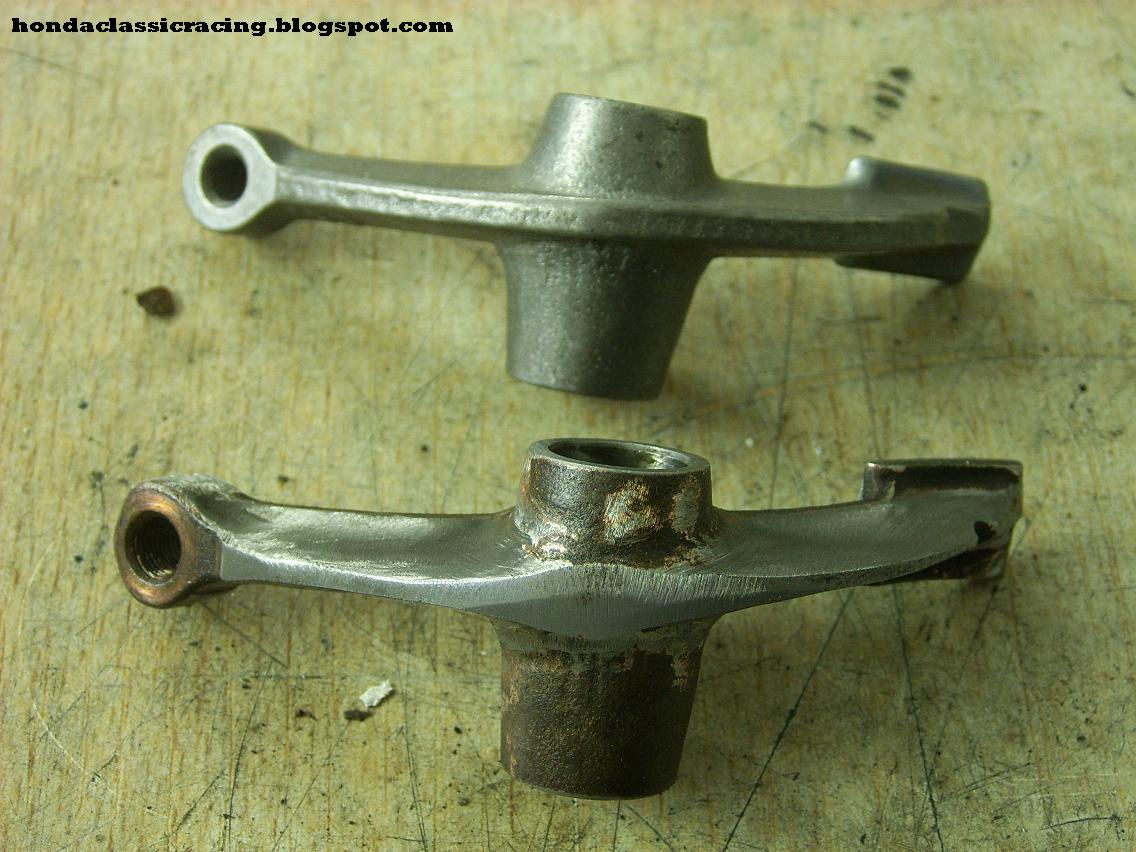This detailed photographic image, set indoors, showcases two metallic components presumably used in racing cars, placed on a heavily scratched, beige wooden table. The upper left-hand corner of the image contains the text "HondaClassicRacing.blogspot.com." The image predominantly features the components placed one above the other, yet they are not connected. Each component begins with an eyelet on the left end, transitions into a curved member housing a cylindrical section in the middle, and ends with a flat tab. Both components are silver-colored; however, the top one appears new with minor gouges on its cylinder, while the bottom one shows significant wear with rust and a yellow sheen on its eyelet. The detailed close-up of these components, coupled with the worn table background, gives a clear contrast between the new and used states of these seemingly identical objects.